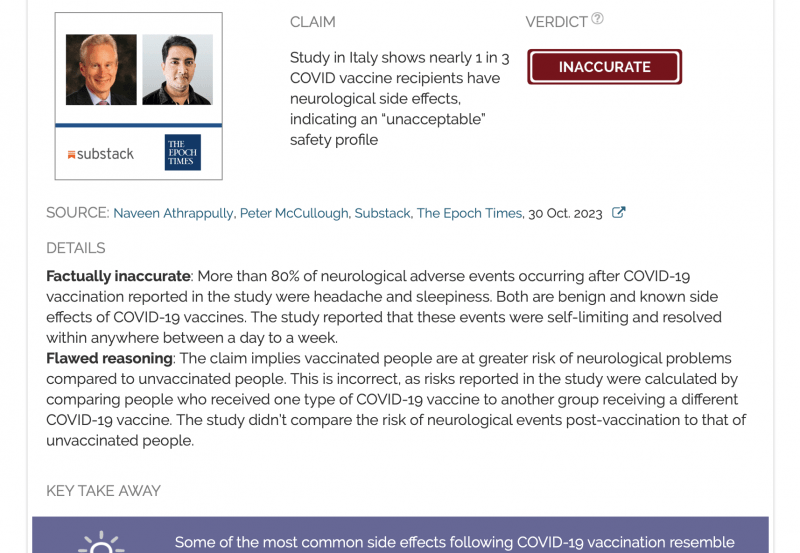The image is a screenshot from a fact-checking website dedicated to verifying and debunking various claims. On the right side of the website, there is a section featuring two profile photos side by side: the photo on the left shows a white man labeled "Substack", while the photo on the right shows a man of indeterminate ethnicity with dark hair, labeled "The Epoch Times". Below these photos, the text reads: "Source: Naveen Athropouli and Peter McCullough, Substack, The Epoch Times, October 30th, 2023."

In the details section, the website highlights in bold the claim, stating it is factually inaccurate: "More than 80% of neurologically adverse events reported after COVID-19 vaccination in the study were headaches and sleepiness. Both are benign and known side effects of COVID-19 vaccines. The study reported that these events were self-limiting and resolved within anywhere between a day to a week."

Further below, another section titled "Flawed Reasoning" explains that the claim implies vaccinated individuals face a greater risk of neurological problems compared to unvaccinated individuals. This is incorrect because the risks reported in the study were calculated by comparing individuals who received one type of COVID-19 vaccine with those who received a different COVID-19 vaccine. The study did not compare the risk of neurological events in vaccinated people to that in unvaccinated people.

At the bottom, a large red button displays the verdict "Inaccurate." The claim being debunked states: "Study in Italy shows nearly one in three COVID vaccine recipients have neurological side effects, indicating an unacceptable safety profile." The fact-checking website debunks the claim made by the right-wing website, clarifying that the assertion about the COVID-19 vaccine's safety profile is false.